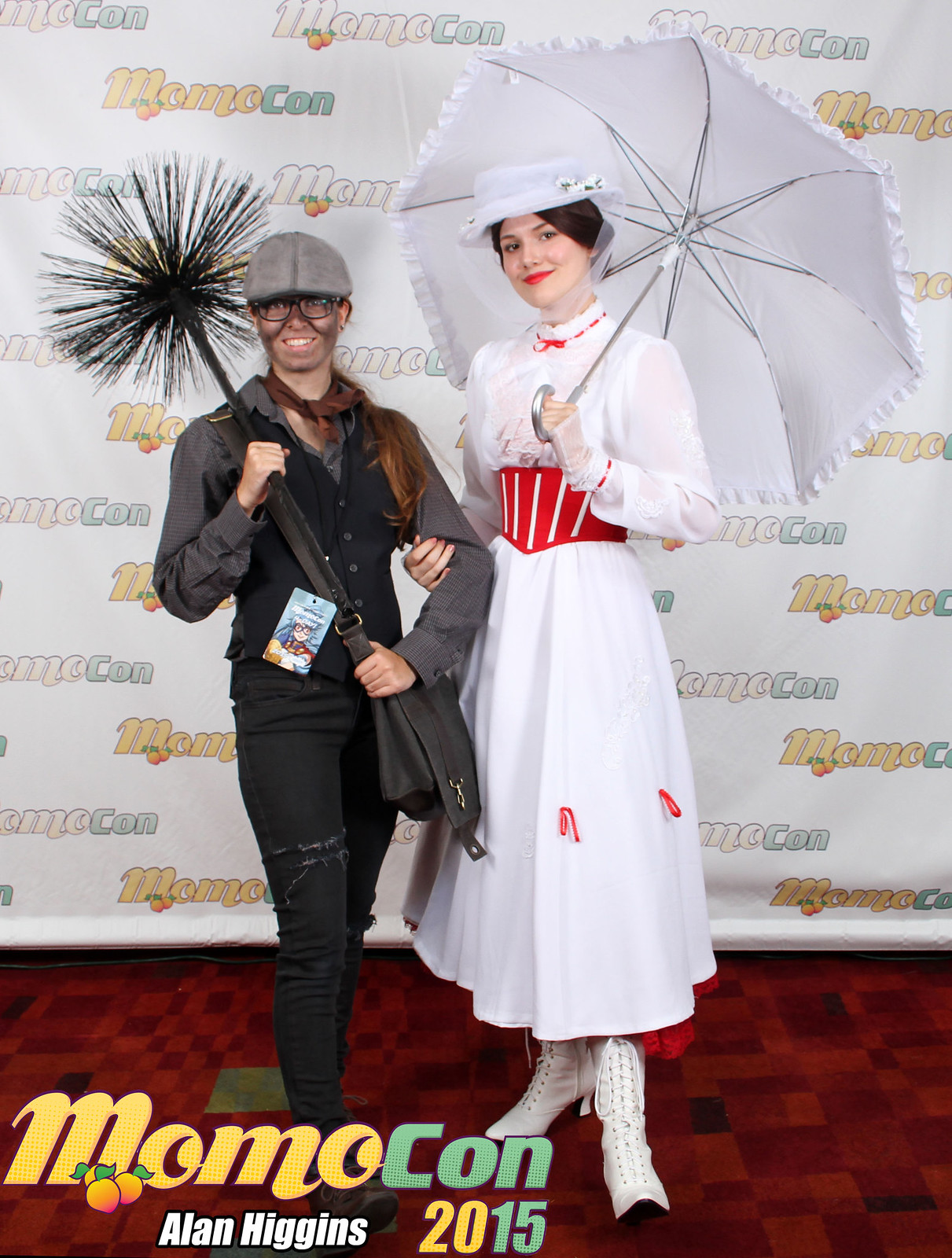The image depicts two women in costume, standing in front of a step-and-repeat backdrop that reads "MOMOCON 2015" in orange and green with a larger version of the logo in the bottom left corner along with the name Alan Higgins. The woman on the left is dressed as a chimney sweep, wearing dark pants, a dark gray collared shirt, and a dark vest. She accessorizes her look with a newsboy cap, glasses, and has dirt smudged on her face to complete her character. She holds a chimney sweep pole and has long red hair. The woman on the right is dressed as Mary Poppins, featuring a white dress adorned with a wide red belt and white boots. She wears a white hat secured with a tulle chin strap and holds a white parasol. Her outfit is further detailed with red accents, including a thick red waistband and red threading around the bottom of her skirt. Both women vividly bring characters from the movie Mary Poppins to life, perfectly themed for the MOMOCON convention.